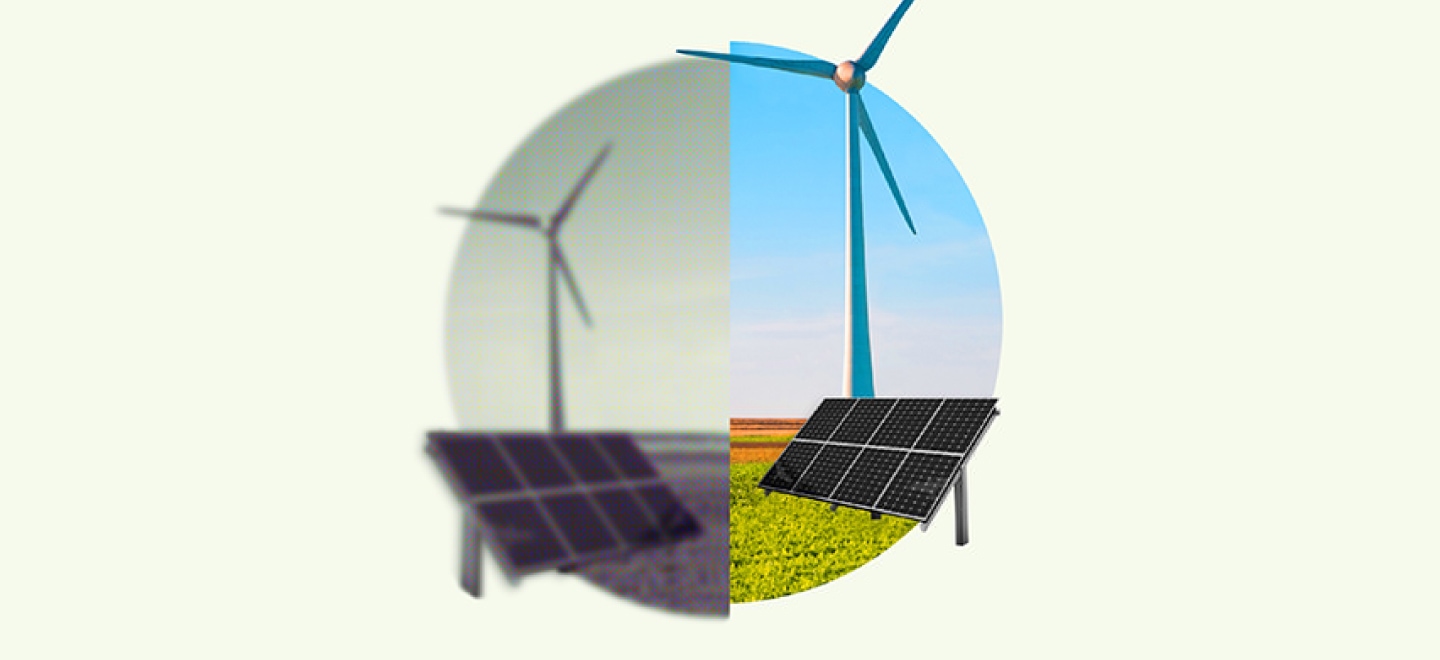The image depicts a centrally-placed circle that is bisected into two mirrored halves, each containing a detailed landscape featuring renewable energy sources. On the left side, the image is blurred and presented in black and white, showing an eight-panel solar array with distinct black panels featuring white dots. Adjacent to the panels stands a wind turbine with three slender blades. The backdrop consists of green grass, orange dirt, and a bright sky, all in grayscale. Contrastingly, the right side showcases the same scene in vivid color, where the blue sky enhances the visual appeal. The wind turbine appears white, and the solar panels retain their black and silver coloring. The green grass below and the brown farming fields in the background add a naturalistic touch to the image. Overall, the juxtaposition of the blurred monochrome left side with the clear, colorful right side provides a striking visual comparison of the same renewable energy landscape.